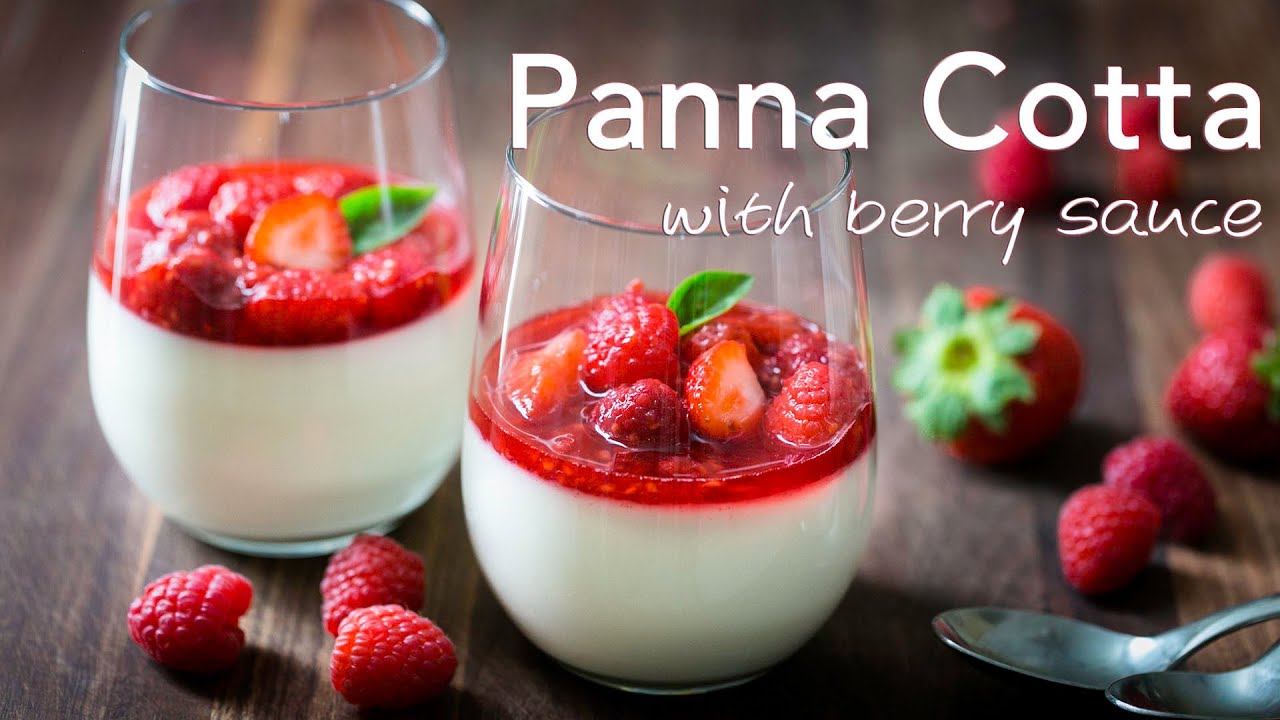This image showcases a delectable serving of panna cotta with berry sauce, labeled clearly in the top right corner in white text with "panna cotta" in a bold, serif font and "with berry sauce" in an informal, cursive font. The panna cotta is served in two crystal-clear stemless wine glasses, each filled halfway with a smooth, white, milk-like substance that is the panna cotta. On top, a half-inch-thick layer of vibrant red berry sauce, dotted with strawberries and raspberries, adds color and texture to the dessert. The glasses sit on a dark wooden table alongside two spoons, with three loose raspberries in front. In the background, slightly out of focus, are additional strawberries and raspberries, enhancing the fresh, fruity appeal of the presentation. A mint leaf garnish adorns the top of the berry sauce, completing this elegant and appetizing display.